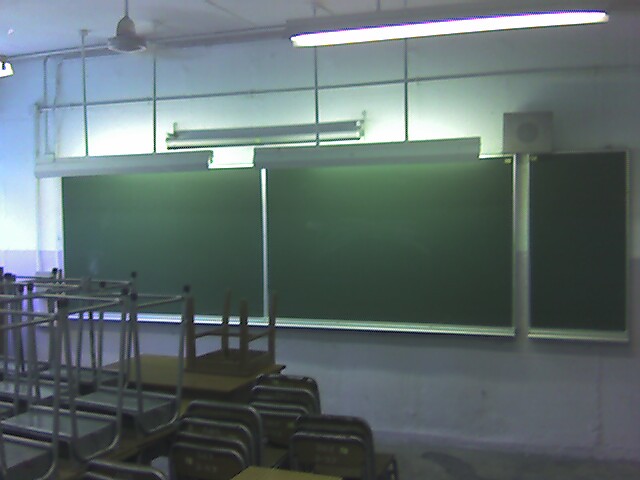The image depicts an empty classroom with distinct features that suggest it is not currently in use. Dominating the front of the room are three green chalkboards—two long and rectangular and one smaller but equally tall, possibly about 10 feet high, providing ample space for writing. Overhead fluorescent lights illuminate both the classroom and the chalkboards, enhancing visibility irrespective of the time of day. Additional lighting fixtures directed at the chalkboards ensure they are well-lit.

In the background, a speaker system is installed on one of the white walls, above which a pattern made of pipes or bars runs across the top. A pull-down movie screen is mounted above two of the chalkboards, although it is retracted in this image. The floor space in the foreground is cluttered with a large, haphazard pile of desks and chairs, some stacked on top of each other and others grouped together, emphasizing the abandoned or temporarily unused state of the classroom. There are no visible chalk or erasers, adding to the sense of disuse. Overall, the scene presents a typical wide-angle view of a classroom awaiting its next session.